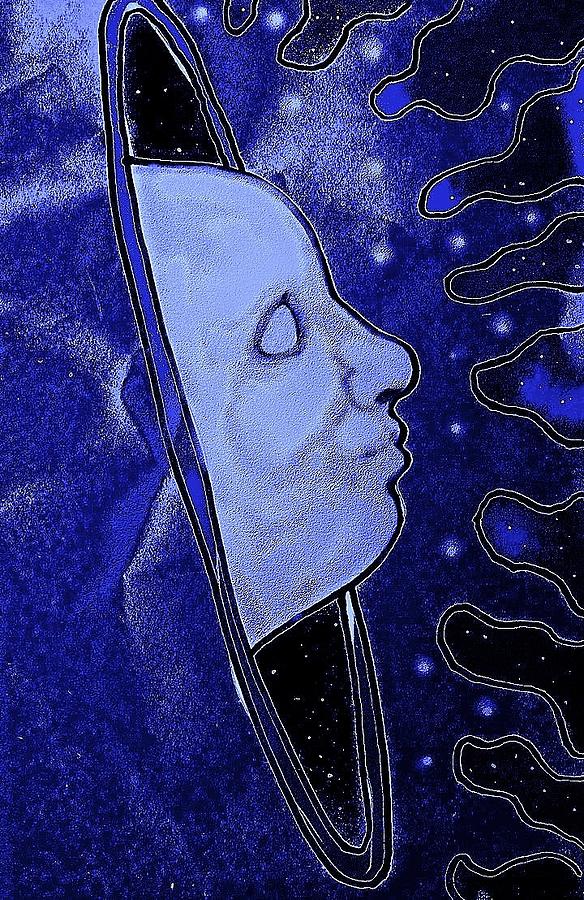This detailed artwork, predominantly in shades of blue, portrays an ethereal scene set in outer space. A black hole or circular portal is centrally featured, flanked by a multitude of lighter colored stars and potential galaxies. Emerging from the blackness of this hole, a hairless and pensive human face of a lighter blue hue peers outward, with blank eyes and minimal facial features. Encircling the face is a radiant blue ring resembling sun rays or flaming tendrils, blending into the surrounding cosmic expanse. The outer regions of the image, which transition back into the star-speckled void of space, emphasize the mesmerizing and otherworldly essence of the scene.